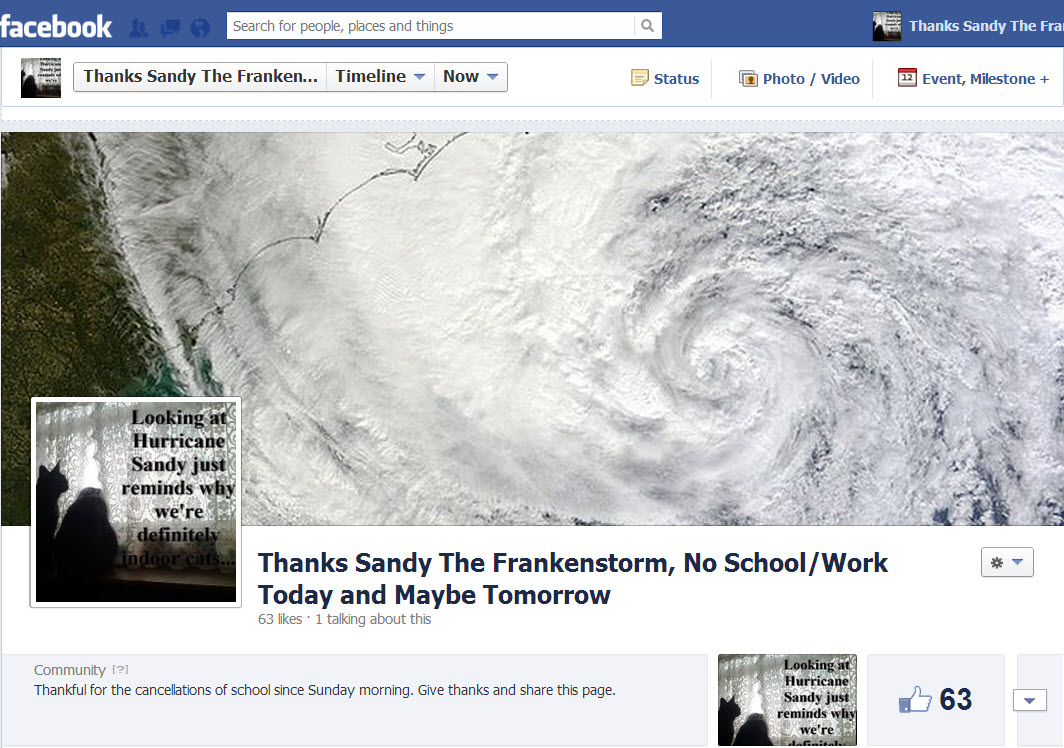In the image, we are looking at a Facebook post on a standard Facebook page layout. The top banner is blue with the Facebook logo on the left side. The logo features the word "Facebook" in white font and an icon of a person’s head in darker blue. In the search bar, a grey magnifying glass icon is positioned to the right of the text "Search for people, places, and things." To the far right, there is white text reading "Thanks Sandy the Fra" accompanied by a user’s profile.

Central in the post is a black and white image of Hurricane Sandy, characterized by a distinct white swirl indicating the hurricane's eyewall, with grey clouds extending outward. Below the image, the text reads "Thanks Sandy the Franken...," fading out. Underneath, there is a grey bar with options: "Timeline" accompanied by a downward arrow, and a similar line for additional options with another downward arrow. These elements are set against a white background.

To the right of the grey bar, there are icons and text options: "Status" illustrated by a yellowish note icon, "Photo/Video" with an icon of two digital photos, and "Events" marked by a calendar icon. Another section reads "Column Milestone Plus."

Below the main image, the caption reads: "Look at Hurricane Sandy; it just reminds why we're definitely..." before fading off. Further commentary states: "Thanks Sandy the Frankenstorm, no school/work today and maybe tomorrow." This is followed by engagement statistics: "63 likes, 1 talking about this."

At the bottom right, there is a grey text reading "Community?" with an encouragement to "Give thanks and share this page." The same hurricane image appears again, repeating the cut-off text, "Look at hurricane Sandy, just reminds why we're..."

Icons for interaction include a grey thumbs-up icon with "63" likes next to it, and partially visible grey boxes with arrows indicating further options or settings. The entire layout maintains Facebook’s trademark clean and structured design.